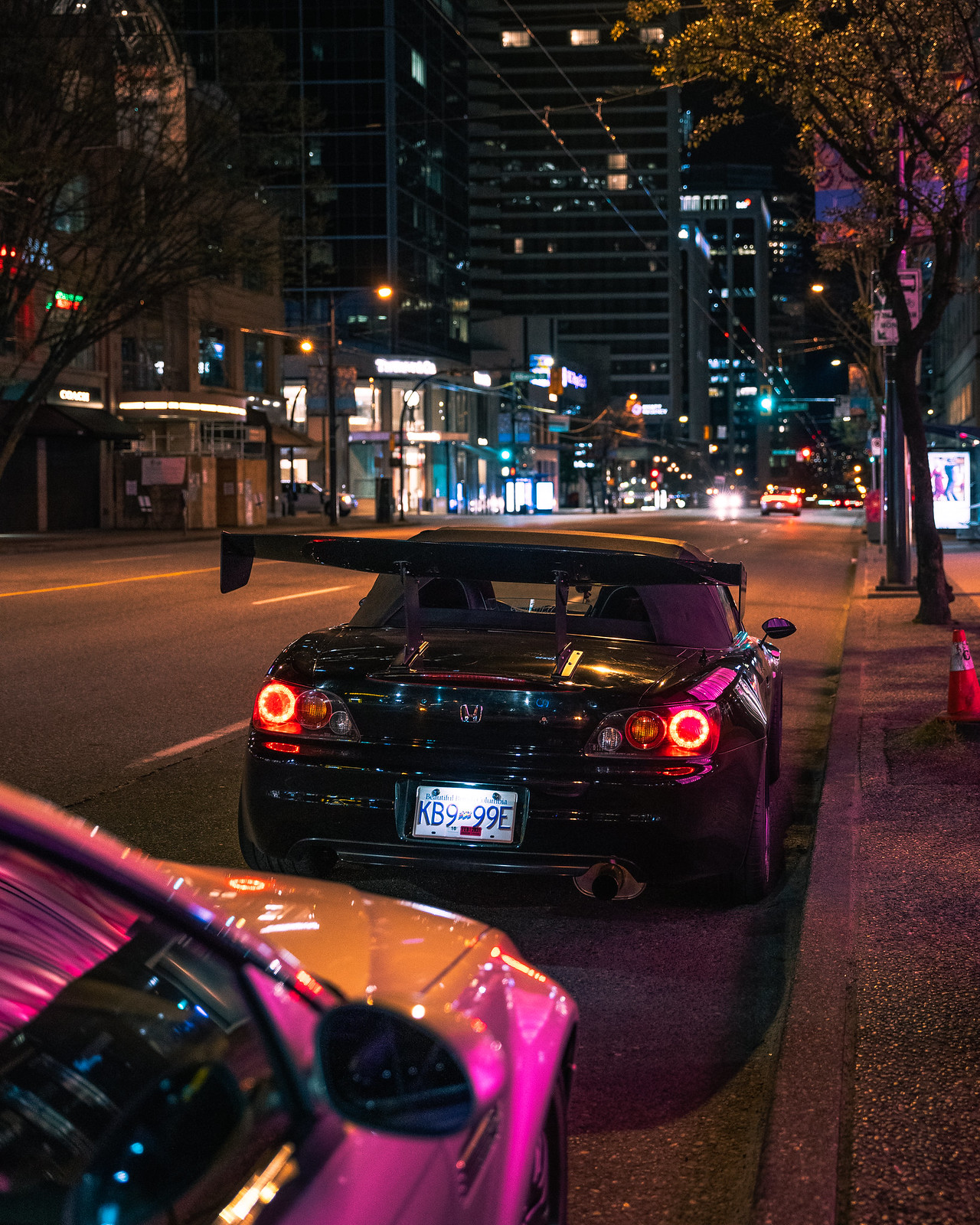This vertical rectangular photograph, taken at night on a city street, showcases a dramatic scene illuminated by streetlights, casting an orange hue on the two lanes of traffic. Prominently in the foreground on the right side of the road is a shiny black sports car, distinguished by its large spoiler and visible license plate KB 999E, with its rear lights glaring. Directly in front of it, almost head-to-head, is a light-colored car—perhaps pink or white—reflecting vibrant hues from the surroundings. These cars seem oddly positioned, as if parked or ready to drive, suggesting a potential misalignment or confusion about the lane directions. The scene extends into a backdrop of distant traffic and a bustling yet sparsely populated cityscape marked by towering skyscrapers and shorter shops, their lights brightly illuminating the night. Trees adorned with holiday lights line the sidewalks, adding a festive touch to this urban tableau, while the absence of pedestrians underscores the stillness of this nocturnal moment.